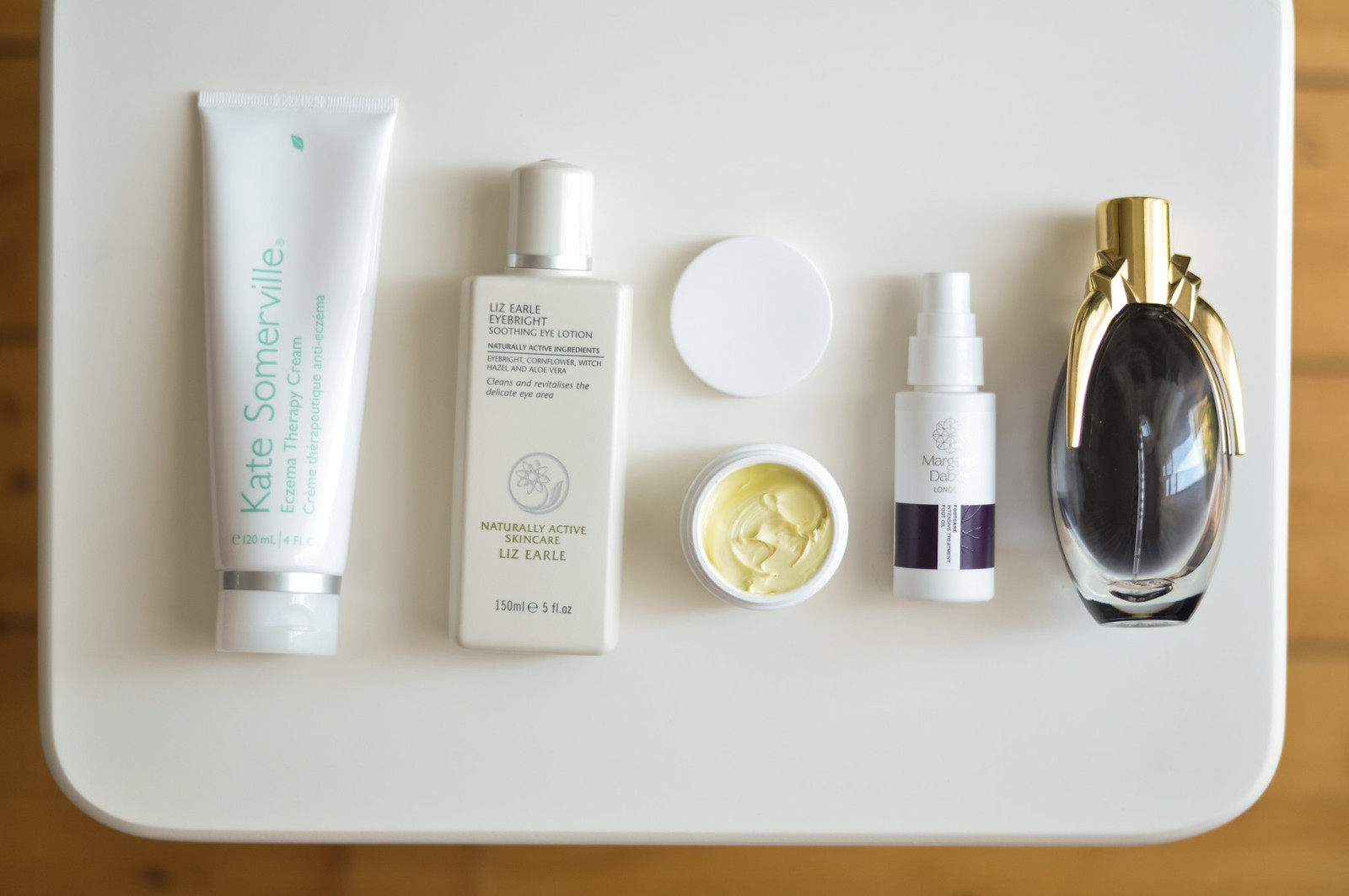The image features a meticulously arranged flat lay of various cosmetic products and perfumes displayed on a white surface, possibly a table or cutting board, set against a wooden floor background. 

1. The first item is a white tube featuring green teal text that reads "Kate Somerville Eczema Therapy Cream," along with additional specifications and the volume in ounces. The tube is elegantly accented with a silver trim around the cap.
   
2. Next is a white bottle labeled "Liz Earle Eye Bright," noted as a soothing eye lotion. The bottle has black text detailing the product information and includes the volume in ounces.

3. Positioned beside these items is a white tub containing a yellow cream. The tub's lid is removed and placed to the side, offering a clear view of the cream within. The container itself is unmarked with any text.

4. A spray bottle is also included in the arrangement. This product features silver writing and some black squares, but its specific type of product remains ambiguous.

5. Finally, a perfume bottle is displayed, characterized by an opaque glass design with black detailing and a sophisticated gold cap.

Each product is thoughtfully spaced to create a visually pleasing composition, highlighting their design and features against the neutral background.